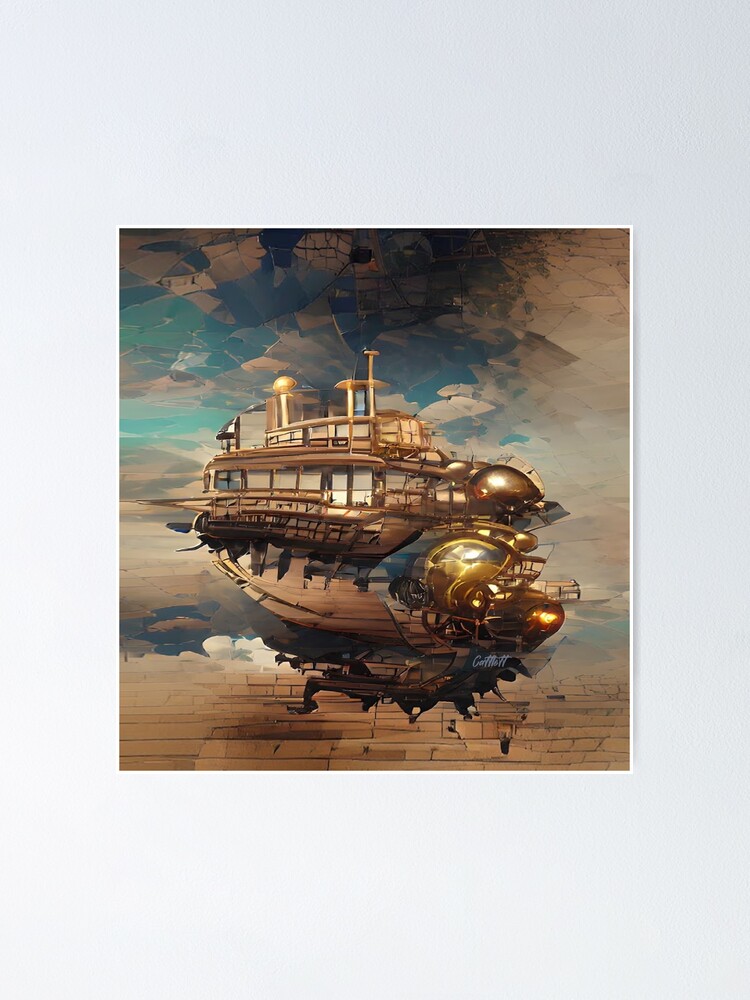The image depicts a surreal, futuristic vehicle that combines elements of a ship, an aircraft, and possibly even a train. Its central structure, resembling a ship's hull, is mounted on a flying platform adorned with glowing lights, glass panels, and a brassy metal reflection. The vehicle features various levels and windows, and a peculiar piece, possibly a propeller, extends from its rear. The background consists of a fragmented blue and white sky, giving an impression of both clouds and shattered glass. Below, what appears to be a brown field segmented into rectangular parcels subtly contrasts the light textures of the sky. The painting, done in a light, watercolor-like style, adds to the overall surreal and fantastical atmosphere of the scene.